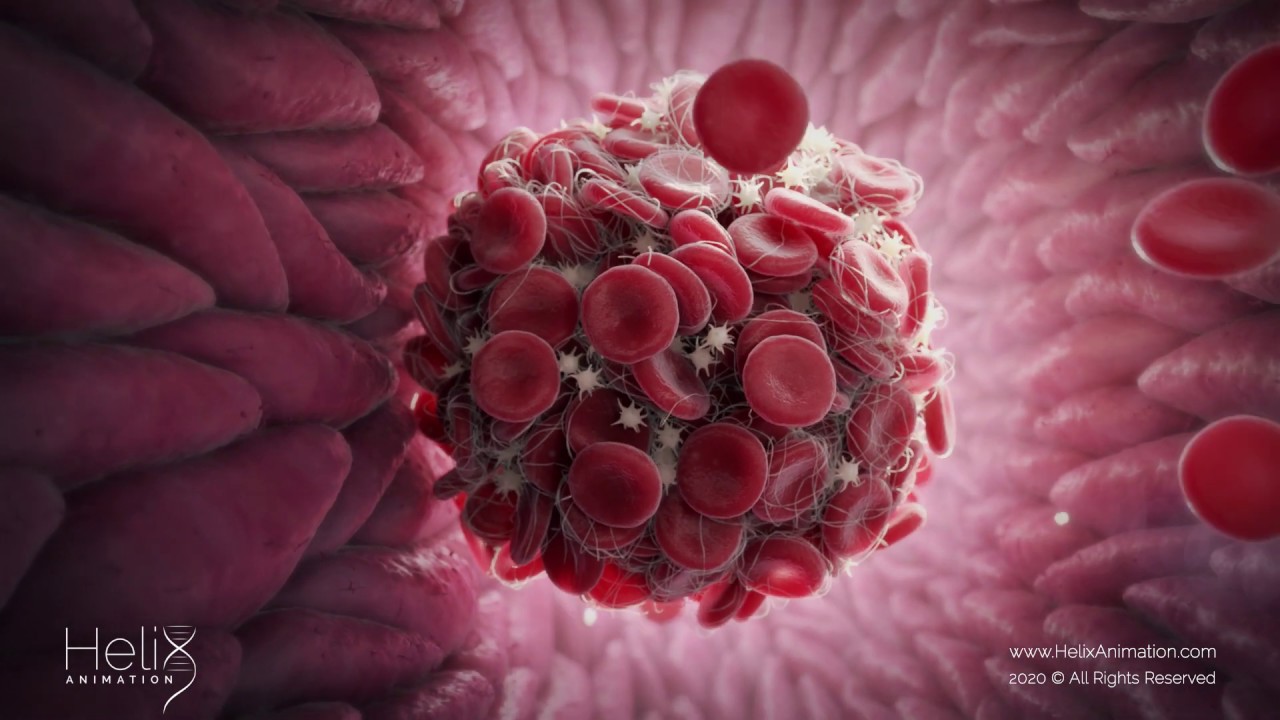The image is a detailed 3D render illustrating the inside of a blood vessel during the formation of a blood clot. At the center of the composition, an aggregation of blood cells and platelets forms a substantial and intricate ball, vividly demonstrating the clotting process that occurs when an injury takes place. The red blood cells, appearing as flat, reddish disks, are intricately bound together by thin, web-like white fibrin threads, while smaller white platelets with spiky protrusions intersperse among them. The background features thick, pillowy, reddish-pink walls, emphasizing the vessel interior, with more red blood cells moving in from the right towards the forming clot. The scene is rich in red and violet hues. In the bottom left corner, the label "Helix Animation" appears, with the "X" fashioned into a double helix shape, and the bottom right corner reads "www.helixanimation.com 2020 copyright, all rights reserved" in white text, indicating the animation's creation and ownership details. The image expertly combines scientific visualization with detailed artistry to depict this essential biological process.